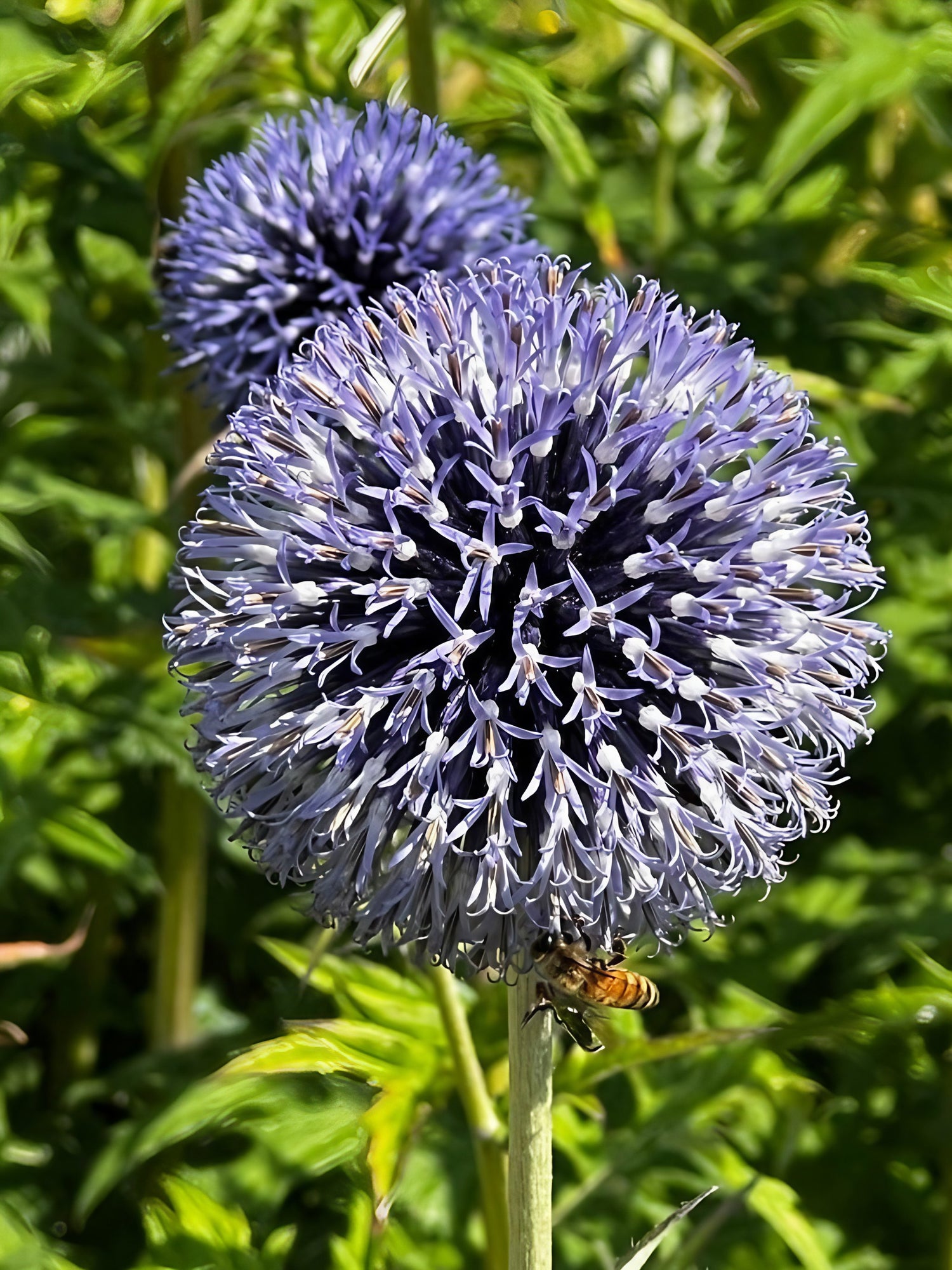This color photograph, in portrait orientation, captures a striking wildflower in full bloom, set against a blurred green background of other plants and shrubbery. The main subject is a spherical cluster of small, purple blossoms, each with delicate four-point petals and a darker, almost bluish-purple core. These blossoms emerge from a dark, bulb-like base at the end of a vertical green stem, which is prominently featured from the bottom center of the image. The floral sphere is meticulously detailed with tiny, white-spiked flowers covering its surface, creating a vivid and textured appearance. Below this primary bloom, a honeybee, recognizable by its gold and black banded stripes, can be seen partially hidden as it crawls up into the flowers, with its wings hanging down and its eyes focused upwards. Behind the main flower, another similar but smaller spherical blossom appears, contributing depth to the composition. The photograph, characterized by its realistic and representational style, provides a well-focused look at the intricate details of the wildflower and the bee, while the background remains softly out of focus to emphasize the central subjects.